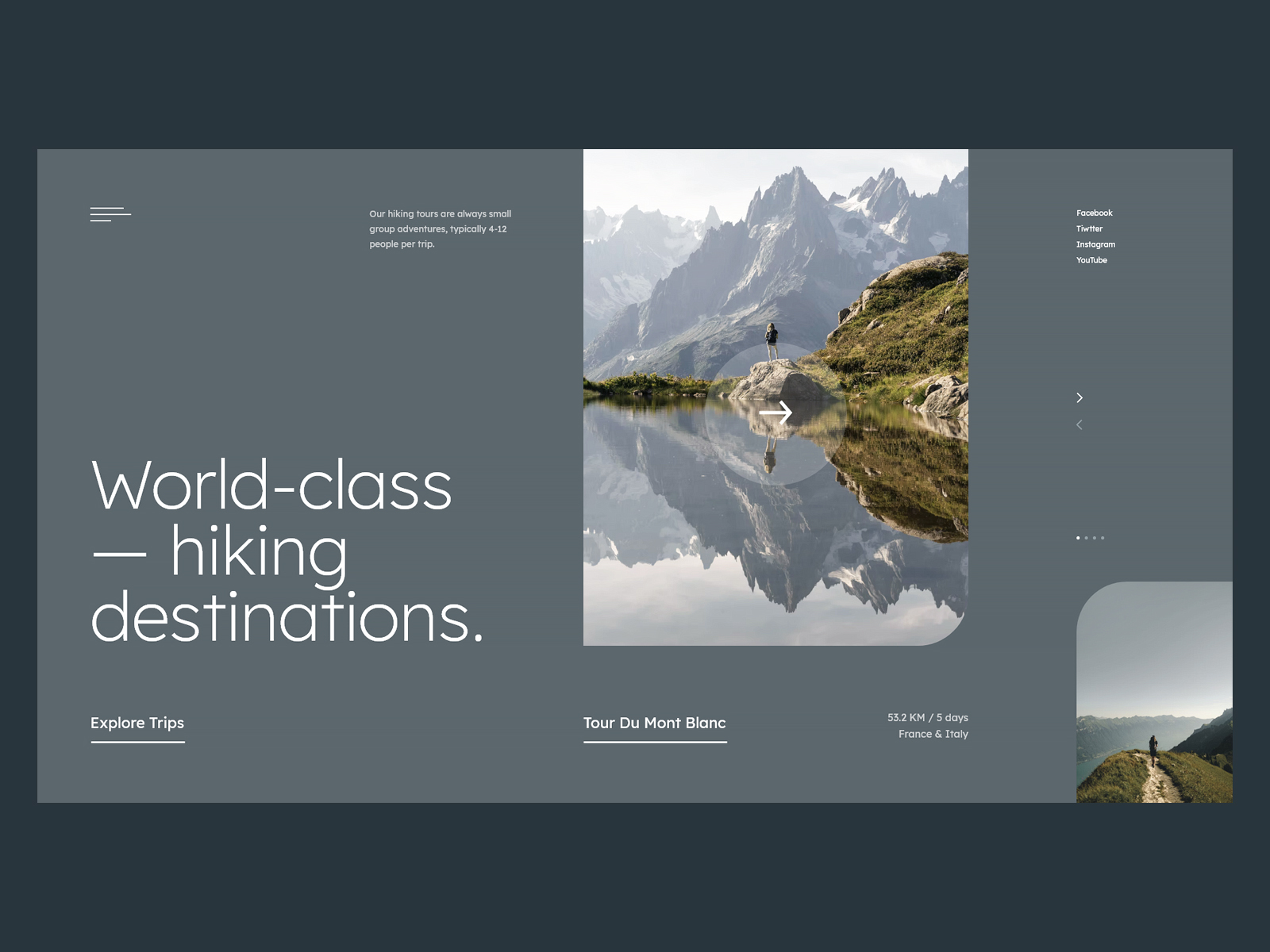A visually striking graphic design or website screenshot features a sophisticated and artistic layout dominated by shades of blue. The backdrop is enclosed by a dark blue border, framing a slightly lighter blue central area. 

In the top left corner, a minimalist three-line icon indicates a dropdown menu. Directly beneath it, bold white letters announce "World Class Hiking Destinations." Below this title, the phrase "Explore Trips" is underlined, inviting further interaction.

Dominating the center of the design is an image of a person standing triumphantly on a rock edge overlooking a body of water. In the background, rugged, snow-capped mountain peaks create a dramatic scene. An arrow on this image suggests that more content can be explored with a click.

Towards the bottom center, the text "Tour de Mont Blanc" is prominently displayed with a clean white underline. In the bottom right corner, a secondary image with rounded corners shows another individual standing on a mountaintop pathway surrounded by lush green foliage, adding to the adventurous appeal of the design.